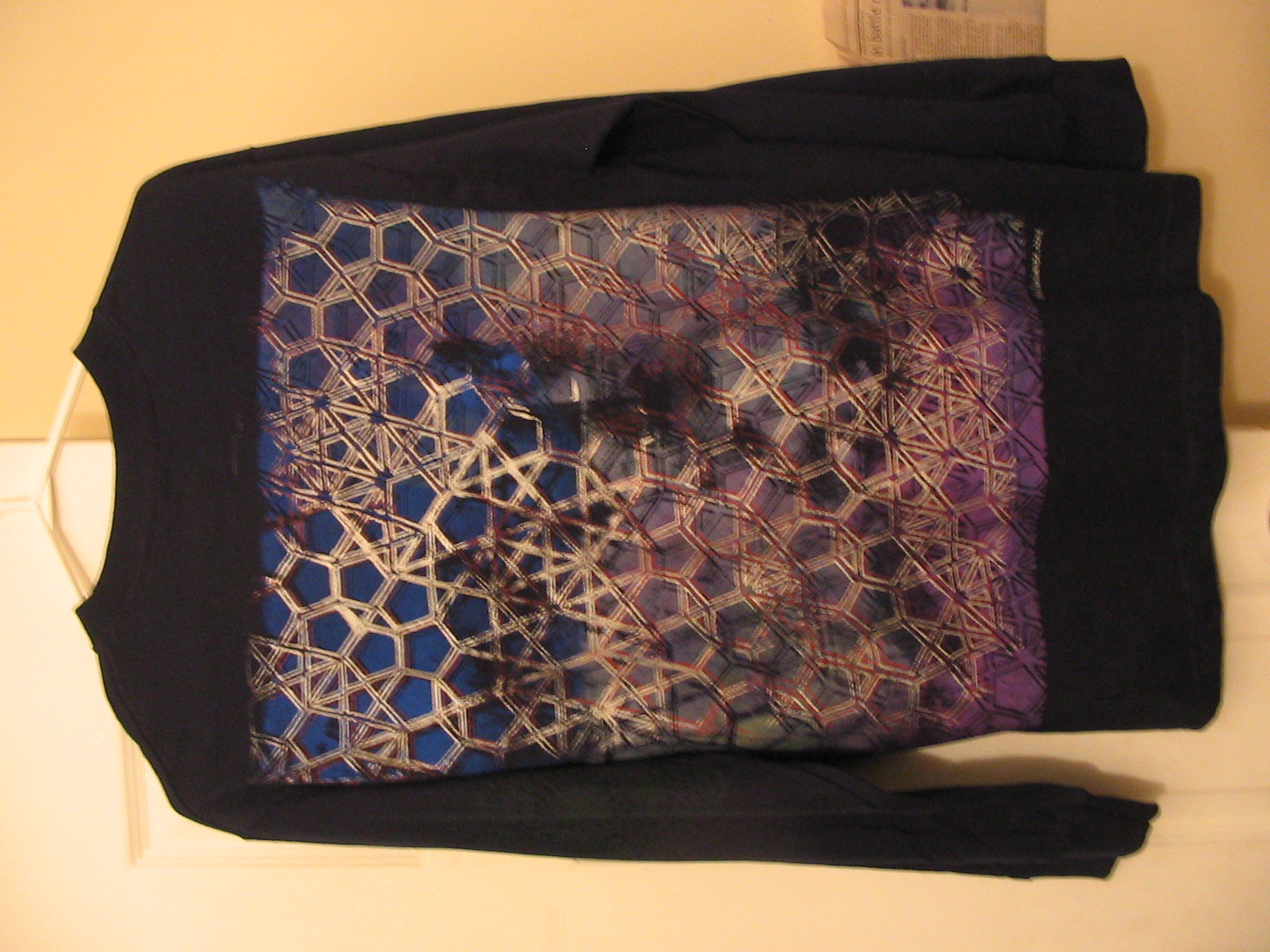A black long-sleeved shirt is displayed on a white hanger, hanging on the corner of a white panel door. The shirt is positioned sideways, showcasing its vibrant front design. The centerpiece of the shirt is a striking logo that spans from just below the collar to nearly the bottom hem. The logo features a gradient background that transitions from blue to purple, adorned with a gold honeycomb pattern interspersed with star shapes. Additional black elements give the design a spray-painted effect, adding an extra layer of visual interest.